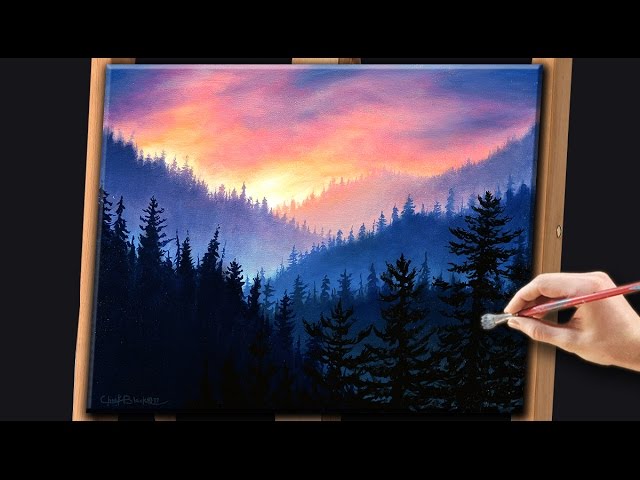The image is a horizontal rectangular photograph of an artist's hand holding a paintbrush, poised to make a touch on a painting displayed on an easel against a black background. The painting itself depicts a vibrant sunset scene in the mountains, with multiple layers of visual depth. In the foreground, there are dark silhouettes of pine trees, transitioning to blue mountains as you move farther back. The sky is awash with an array of colors, including yellows, oranges, pinks, and purples, with dark edges at the top. The painting, which has a signature in the lower left corner, appears to be complete, suggesting the hand might be demonstrating a painting technique rather than actively adding to the artwork. Given the black frames at the top and bottom of the image, it may also be a screenshot from a demonstration video.